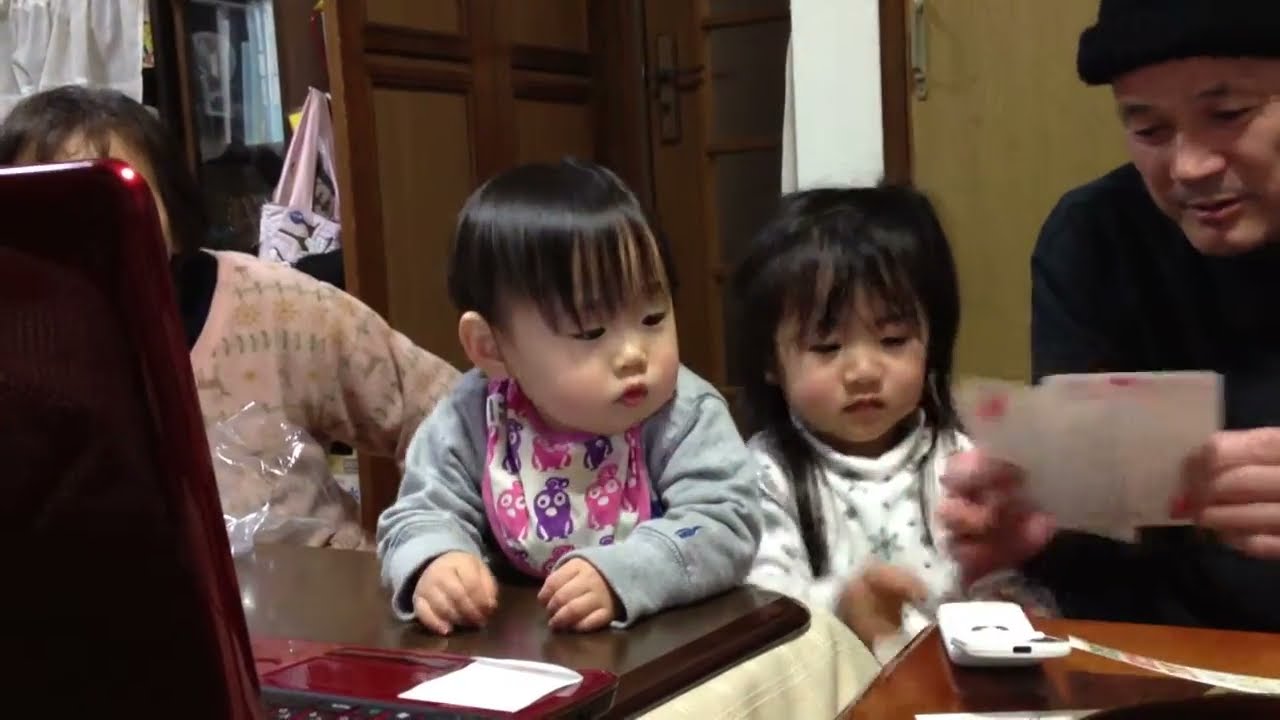The image depicts an Asian family inside a home, centered around two young children. In the middle, a toddler boy with short black hair that almost covers his eyes is leaning against a wooden surface, wearing a gray long-sleeved shirt and a bib adorned with cartoon characters in pink and orange. To his right, a toddler girl with long hair that reaches her chest, possibly in two braids or ponytails, is engaged as both children gaze intently at white cards held by an older man. The man, positioned on the right side of the image, is dressed in black with a beanie and carefully examines the cards in his hands. On the far left, partially obscured by a red panel or open laptop screen, is a woman in a light pink sweatshirt with floral designs, showing only her brown hair and a bit of her face. The backdrop features a brown wooden door flanked by white wall sections, a lighter brown door, and various household items like a pink bag and books on shelving. The setting, decorated in light green hues, emphasizes a cozy, lived-in atmosphere of this familial moment.